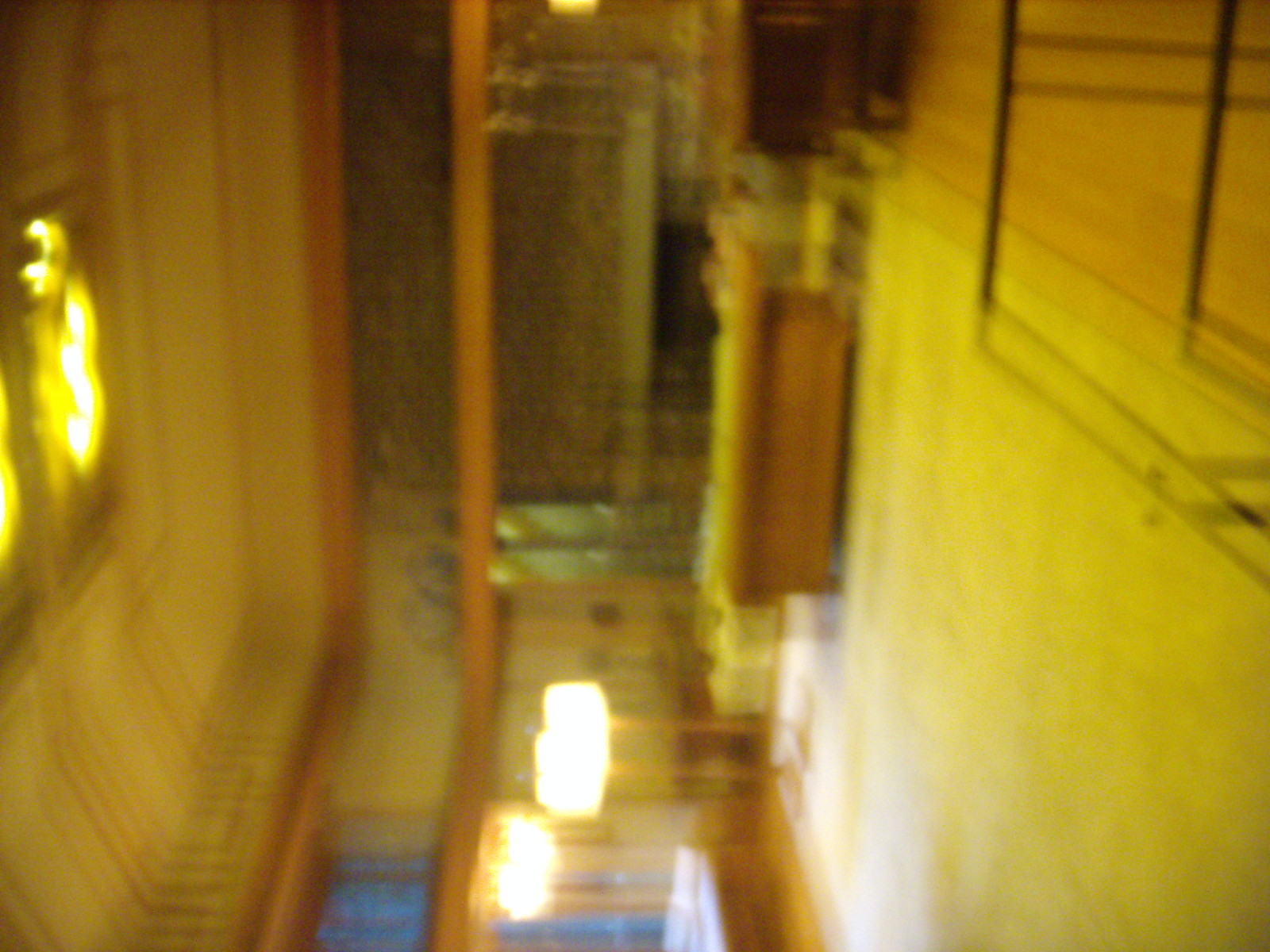This image is a very blurry color photograph that appears disorienting and difficult to interpret due to its tilt and rotation. The scene might be inside a quiet building that could be a bank, museum, or perhaps even a living room. The dominant colors are yellow and beige, lending a slightly warm and dim ambiance, possibly from the overhead and floor lamps that create a soft glow reminiscent of after-hours lighting.

The image seems to tilt sideways, with the ceiling on the left and the floor on the right. The ceiling, which is tan with wooden beams acting as molding, features yellow lights that cast a warm hue throughout the room. A gray structure resembling a fireplace stands out, with a tan sofa positioned in front of it. This sofa has additional objects, such as a couple of floor lamps near it, and next to it, there's a chest of drawers. Despite the blurriness, you can make out the outline of a wire clear glass table and possibly a rope demarcating a line queue area.

Overall, the photograph’s blurriness and rotation make it challenging to discern specific details, leaving only an impression of an empty, softly lit interior space characterized by a yellowish glow and wooden hues. The confusion and disorientation are enhanced by multiple repeated shapes and figures due to the photo's poor focus and awkward angle.